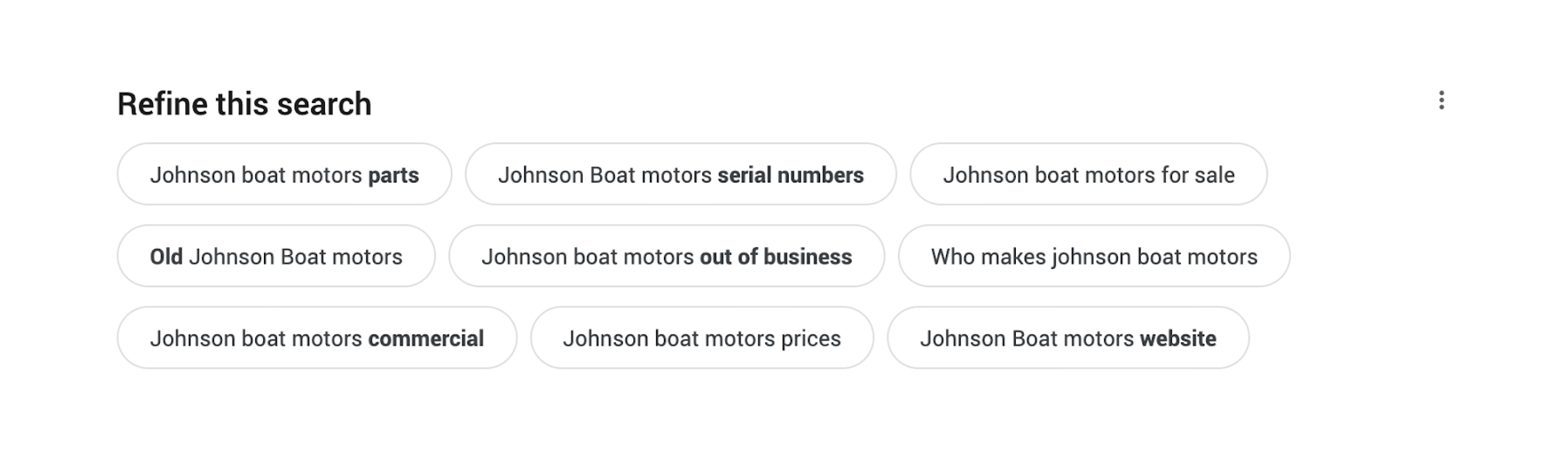A Google search results page featuring a list of refined search options related to Johnson boat motors. The page appears incomplete, displaying only the bottom section with several suggested search refinements in bold. These bolded suggestions include "Johnson boat motor parts," "serial numbers," "older Johnson boat motors," "out of business," "commercial," and "website." There’s a context menu located on the far right of the page. The background is plain white with black text, indicating a possible error or an unfinished search input.